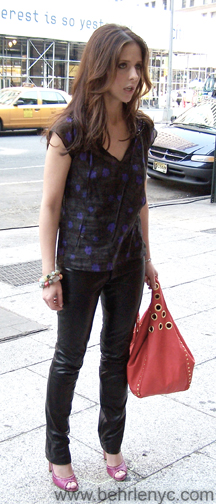A young woman with long brunette hair stands on a sidewalk in a city, positioned directly in the middle of the vertical shot. She faces the right side of the frame, wearing a sleeveless black v-neck blouse with blue spots and tight-fitting black leather pants. Her outfit is completed with red or dark pink peep-toe high heels and gold-riveted bracelets on her right wrist. She's carrying a large coral-colored handbag with gold rivets. Behind her, a partially visible sign on a building reads, "Interest is so yesterday." The background suggests an urban setting, possibly near a car dealership, with several cars and a building featuring a mix of colors including black, white, dark blue, light red, pink, brown, yellow, greenish-blue, and gray. Text at the bottom right corner of the image reads, "www.behrle-nyc.com," implying a casual, candid style reminiscent of a pedestrian or onlooker’s snapshot.